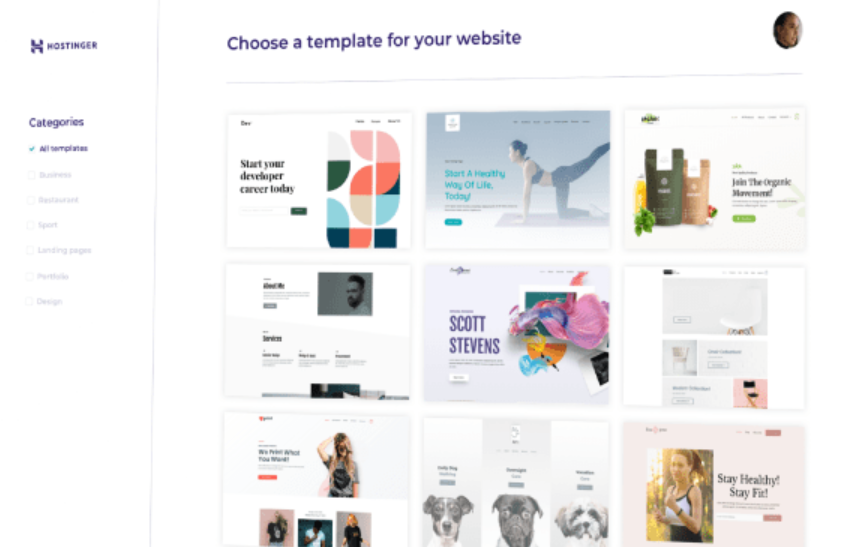The image features a template selection interface from Hostinger. In the upper-left corner, the Hostinger logo is prominently displayed. Below the logo, a header reads, "Choose a template for your website." A small circular profile image is also present near the header. 

The sidebar on the left lists categories, starting with "All Templates" followed by other categories like "Business," "Landing Pages," and more, though some of these are hard to read. 

In the main section, there are nine square preview images displaying different website templates. The top-left template includes a mix of graphics and text, while the second template features a woman practicing yoga. The third template shows bar-like elements. On the second row, the first template appears to be a page layout with various text blurbs, and the middle template prominently displays the name "Scott Stevens." The bottom-middle template features an image of three dogs with text above them. Each square represents a distinct website template option available for selection.